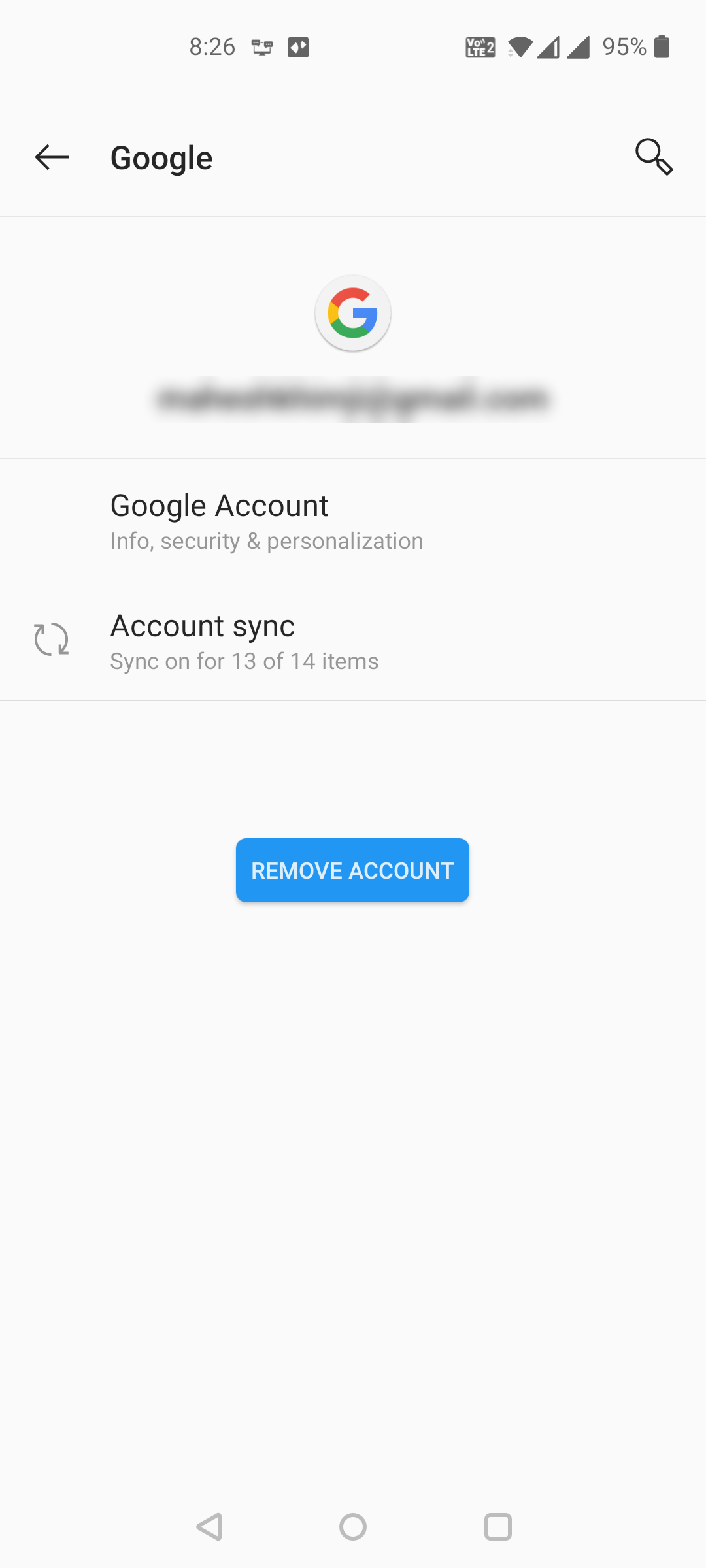The screenshot captures a detailed view of a Google Account sync interface on a computer screen. Dominating the center of the screen is the iconic Google logo. Below the logo, there are two selectable options: "Google Account" in black letters, which offers information about "Info, Security, and Personalizations," and "Account Sync," accompanied by a logo of two curved arrows forming a circle, indicating that syncing is enabled for 13 out of 14 items.

The top of the screen displays a timestamp reading 8:23, alongside several notification icons typical of a tablet device. These icons show a full Wi-Fi signal, a robust telephone signal, and a battery level at an impressive 95% charge. Positioned just below these notifications is a Google search bar featuring the word "Google" in black, a back arrow on the left, and a magnifying glass icon on the right for initiating searches.

At the very bottom of the screen, a prominent blue button labeled "Remove Account" is visible, providing an option for the user to disconnect their account from the device. The overall screenshot provides a comprehensive snapshot of a user's Google Account settings interface with clear indications of account status, syncing details, and device notifications.